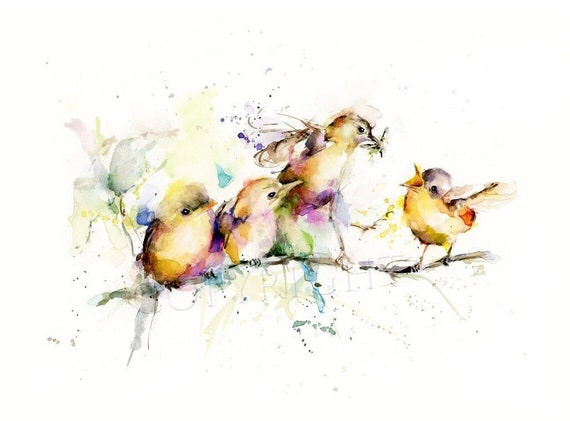This watercolor painting, created on pristine white paper, features a delicate brown tree branch extending from the right side of the composition. Perched on this branch are four vibrant birds, each predominantly adorned in yellow with striking black heads and touches of red on their backs. The two birds on the far right are intently observing a third bird, which is captured mid-flight, ascending with dynamic energy while gazing down at the fourth bird below. This fourth bird, facing its companions with an open beak, possibly awaits food from the flying bird, suggesting a scene of nurturing. The artist adds depth and whimsy with shades of purple beneath the birds, and the painting is further enlivened by a sprinkling of blue, purple, black, and yellow specks, achieved through a flicking technique that adds texture and vibrancy to the composition.